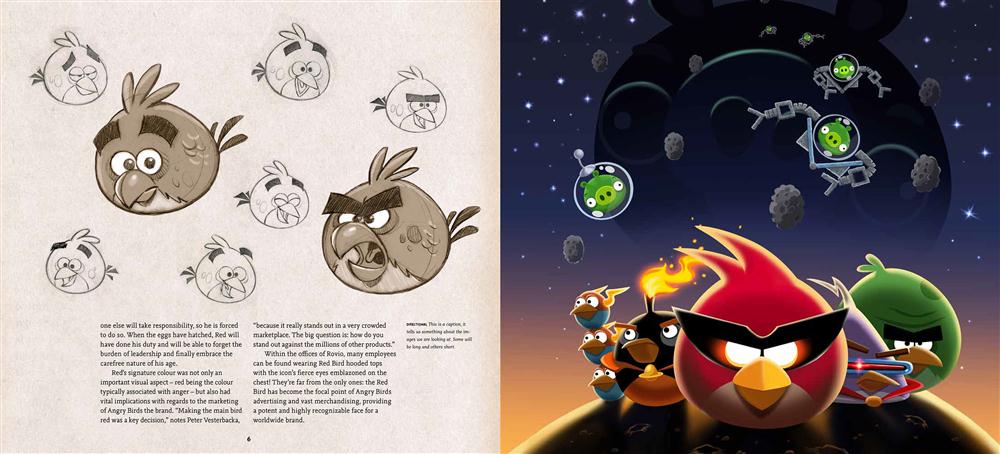The image appears to be a detailed two-page spread from a book featuring Angry Birds characters. The right page showcases colorful, cartoon drawings of various Angry Birds. At the center is the iconic Red Bird, sporting black sunglasses with eyes glowing orange and white on the sides, and a yellow beak. Surrounding him are the three Blue Birds grouped together, a black Bomb Bird with a fiery top, a green bird to the far right, and a Purple Bird with a visor positioned between the Red and Green Birds. The background depicts pigs in astronaut helmets floating in a dark blue, starry sky, suggesting a space theme.

The left page consists of black-and-white sketches of the birds, including repeated illustrations of the Red Bird and another unidentified bird, totaling six images of the latter. Alongside these sketches is small, barely readable text that seems to narrate the creation and characteristics of these characters. Both pages emphasize the spherical, legless design of the birds, characterized by large eyebrows and feathers on their heads and tails.